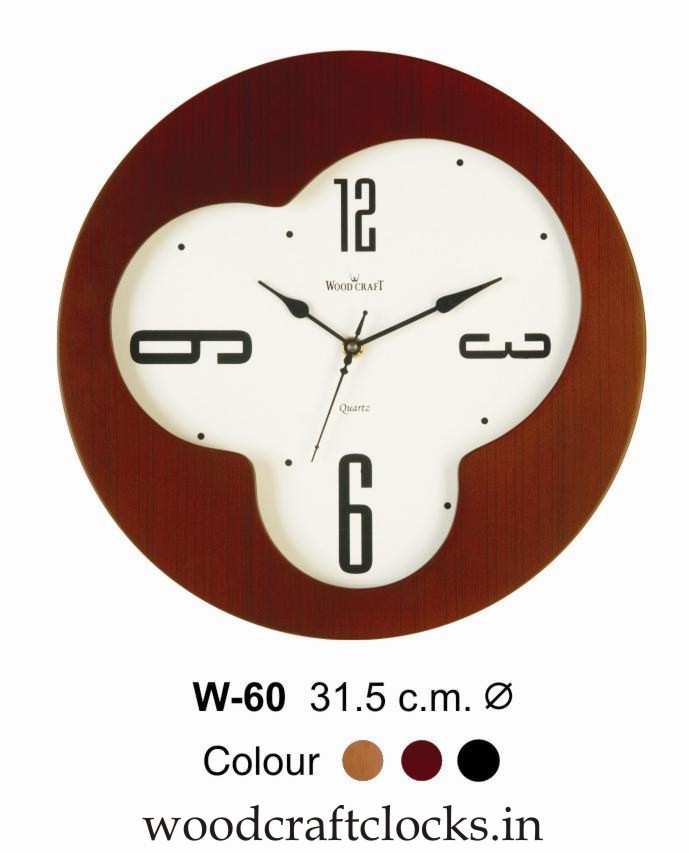This is a detailed, computer-generated image of a wall clock, designed to resemble a photograph. The clock features a brown frame and a uniquely molded face. Only the 12, 3, 6, and 9 are numerically represented on the clock's face. The brand name "Woodcraft" is prominently displayed just below the 12. Below the clock, additional specifications are listed: model W-60, size 31.5 cm, and color options available on the website Woodcraftclocks.in.